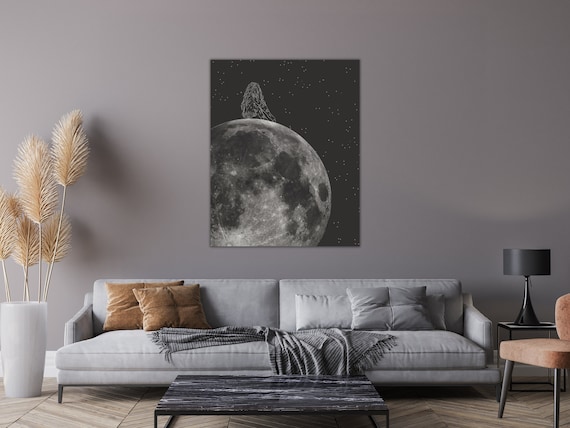This rectangular image captures a well-appointed living room, wider than it is tall. Dominating the space is a long, light gray couch with deep, plush seats, adorned with four throw pillows: two square brown ones on the left and two gray pillows on the right, one of which is rectangular and grayish-white. A darker gray blanket is casually draped in the middle. The wall behind the couch exhibits a gradient from lighter grayish-purple on the left to darker on the right, enhancing the room's visual interest. Centered above the couch is a rectangular picture featuring a space scene, with a large planet on the bottom left corner against a backdrop of stars in a black sky. On the left side of the picture, a ceramic vase filled with tan-colored, feathery stems sits as an accent piece. The room features a wood floor with angled panels. In front of the couch is a low black coffee table. To the right side is a small black side table with a matching black lamp, next to a partial view of a brown chair, adding a warm contrast to the modern, cool color palette of the space.